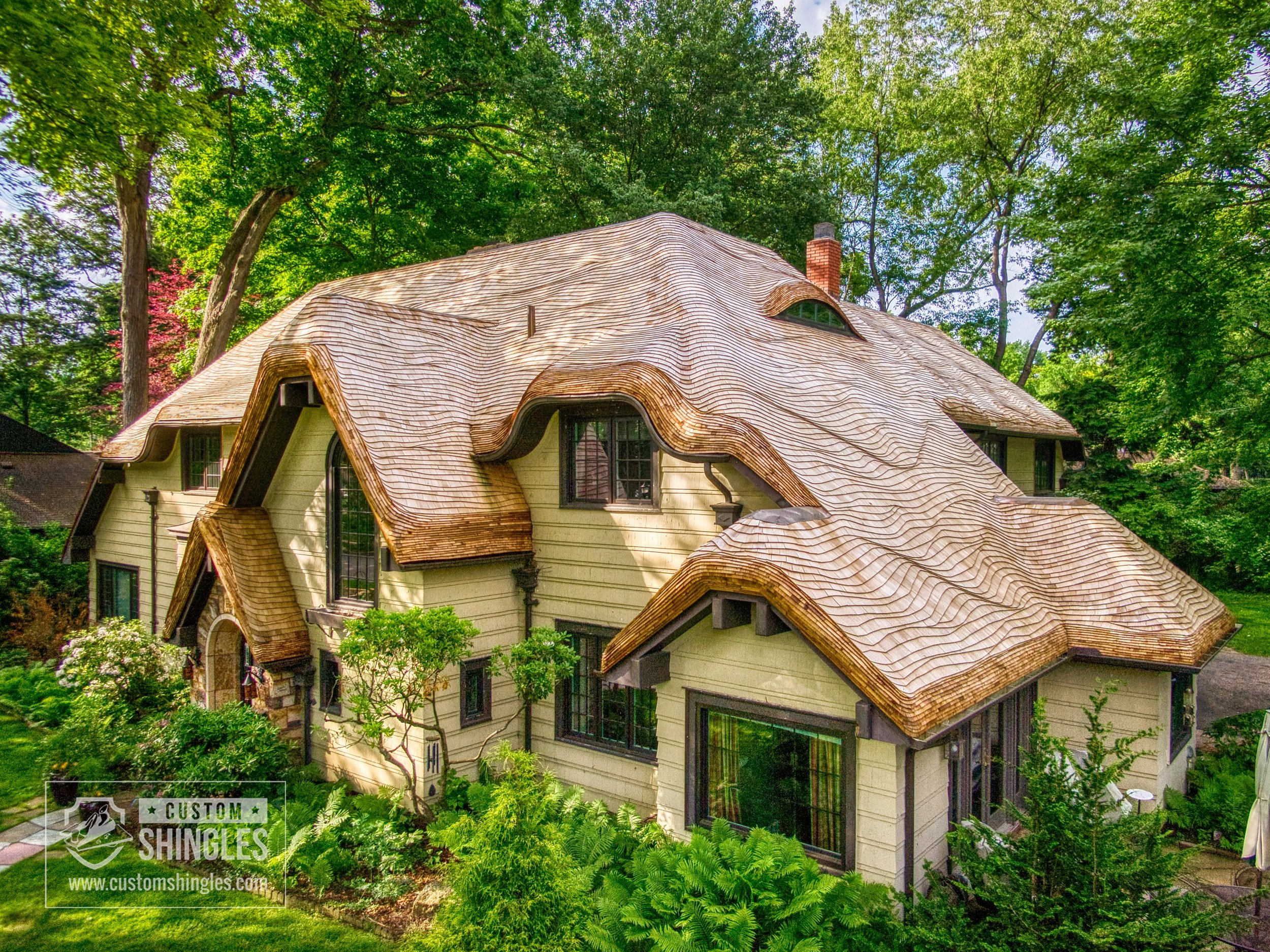The image showcases a uniquely shaped, whimsical home reminiscent of a gingerbread house, set amidst a lush, wooded area with blue sky visible through the trees. The house, designed in a Tudor style with yellow paneling and dark wooden beams, features an imaginative roof with wavy, brown shingles that give a dripping, layered effect similar to the pages of a book or frosting. The shingles' distinctive appearance aligns with the advertisement for Custom Shingles, seen in the bottom left corner with their website. The house itself is surrounded by an array of plants, bushes, and a tree, and partially obscures a brick chimney in the background. Even though the image, likely taken from a mid-tree vantage, prevents a direct view of the front door, an archway leading to it is visible, emphasizing the home's fantastical, almost cottage-like charm. Another house's roof peeks from the left, adding to the serene, wooded setting.